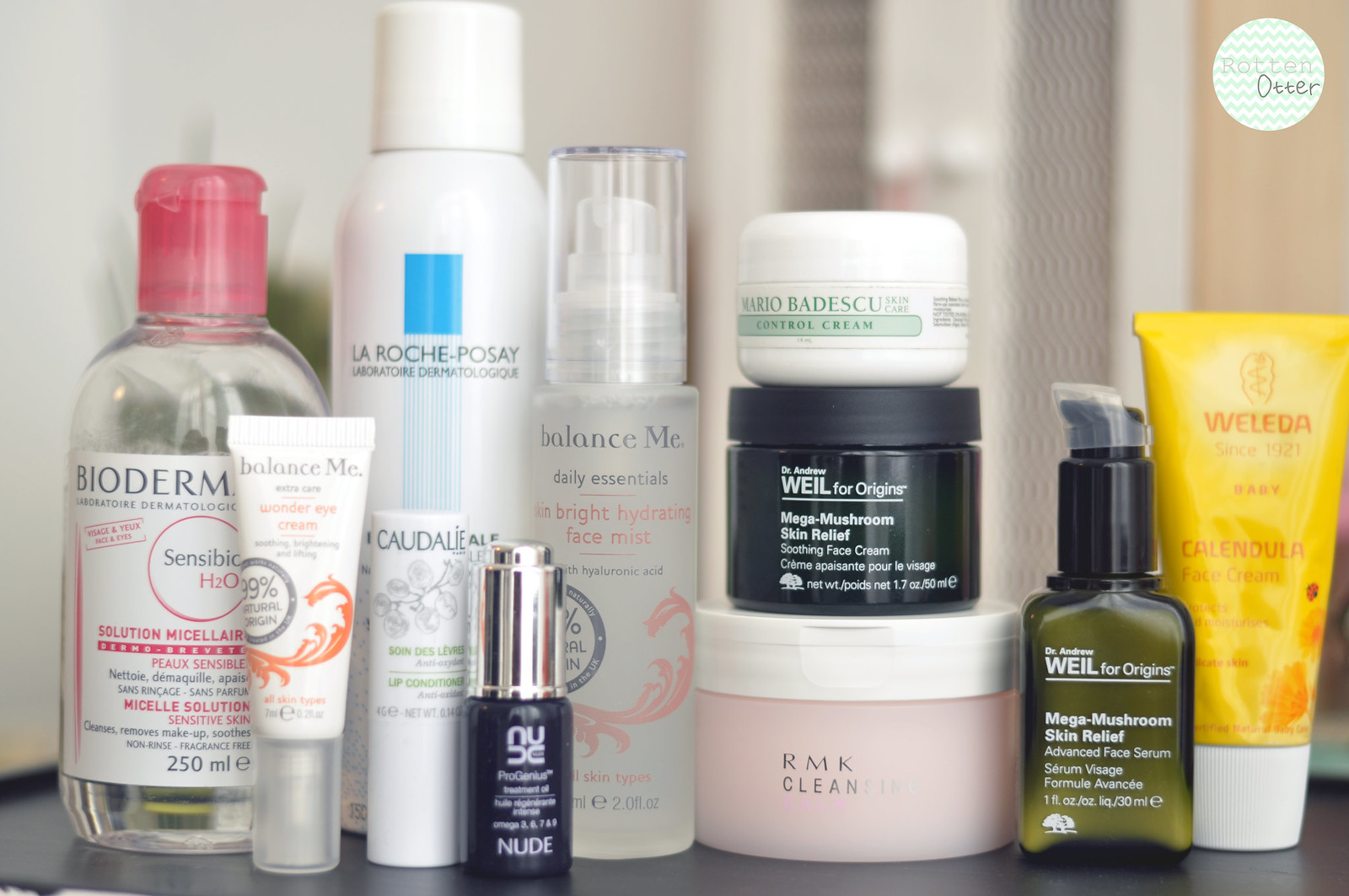In this advertising photograph, a meticulously arranged collection of about 10 or 11 self-care products is displayed on a sleek black table. The background is artistically blurred to focus attention on the diverse array of items. Prominently featured is a small, partially transparent green bottle labeled as Mega Mushroom Skin Relief. Nearby, three squat bottles of varying colors—pink, black, and white—are stacked atop one another, contributing to the aesthetic appeal of the arrangement. Among these, another Mega Mushroom Skin Relief bottle and a Control Cream bottle can be identified.

Additionally, there's a conspicuous tube labeled Balance Me, a clear plastic bottle with a white label branded as Bioderm, and a tall, narrow, opaque white bottle from La Roche-Posay marked with their signature vertical blue rectangle. Completing the tableau is a vibrant yellow tube with a white cap, standing proudly with its inscription, Weleda, indicating it is a face cream. This curated assortment embodies a well-rounded selection of skincare essentials, each product contributing to the overall sense of luxury and care.